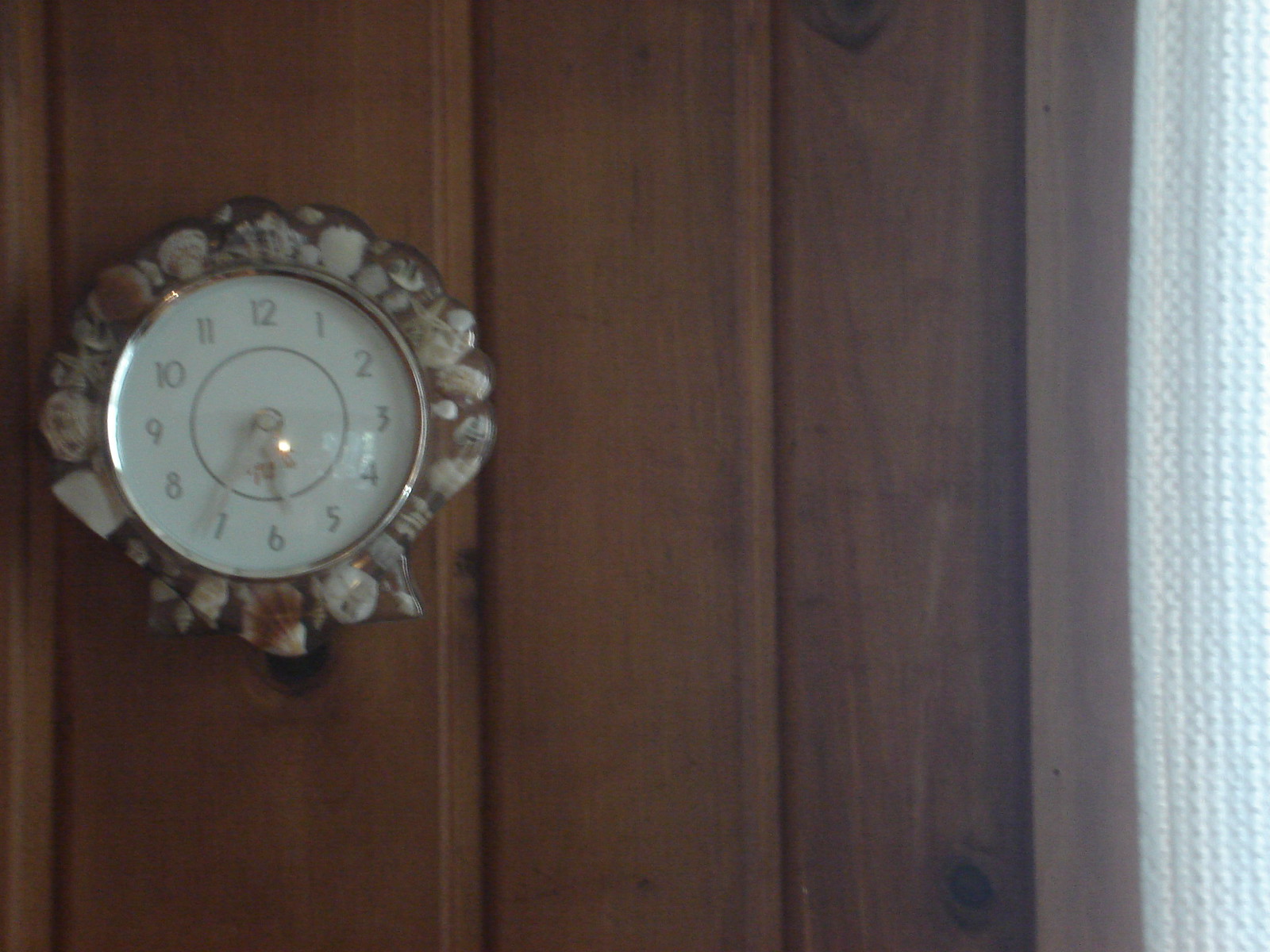This photograph captures a cozy indoor setting, focusing on a distinctive clock mounted on a wooden-paneled wall. The wood panels, composed of vertical planks, are a dark brown hue that adds warmth to the space. In the right-hand corner of the image, a white curtain, textured with lines and possibly made of a rough cotton material, filters in bright light from the adjacent window.

The central feature of the image is a unique circular clock affixed to the left side of the wall. The clock’s face is white, detailed with black numbers ranging from 1 to 12. The hour and minute hands are also black. Surrounding the clock face is a border adorned with an array of seashells in various shades of white and brown, including small clam shells and a tan starfish, all glued onto a brown base, giving the clock a nautical theme. This blend of natural textures and earthy colors creates a visually compelling scene that is both homely and distinctive.